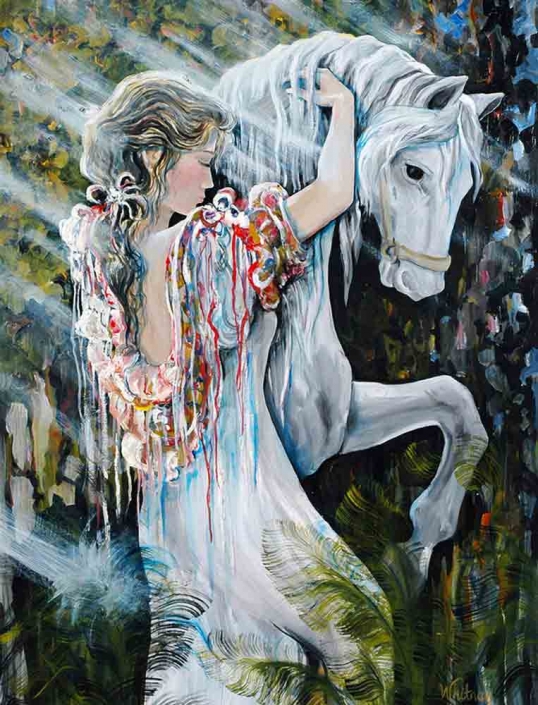This vertical rectangular painting features a serene scene of a young, light-skinned Caucasian woman with blondish-brown hair adorned with flowers, wearing a long, white, flowy dress that has a floral and frilly design around the upper part and drapes down her back. The dress has a unique appearance with colorful paint-like patterns dripping downwards. She stands intimately close to a majestic white horse with a long, flowy mane that subtly incorporates blue hues. The woman gently hugs and pets the horse, her eyes closed, and her head resting on the horse's neck, capturing a tender moment. The horse, adorned with a white bridle, stands with one leg bent and its head slightly lowered. The background is artistically abstract, blending greens, blues, and whites to evoke a sense of sunlight shining through a lush, green landscape with a blue sky overhead. Greenery at the bottom of the scene adds to the natural and tranquil atmosphere.